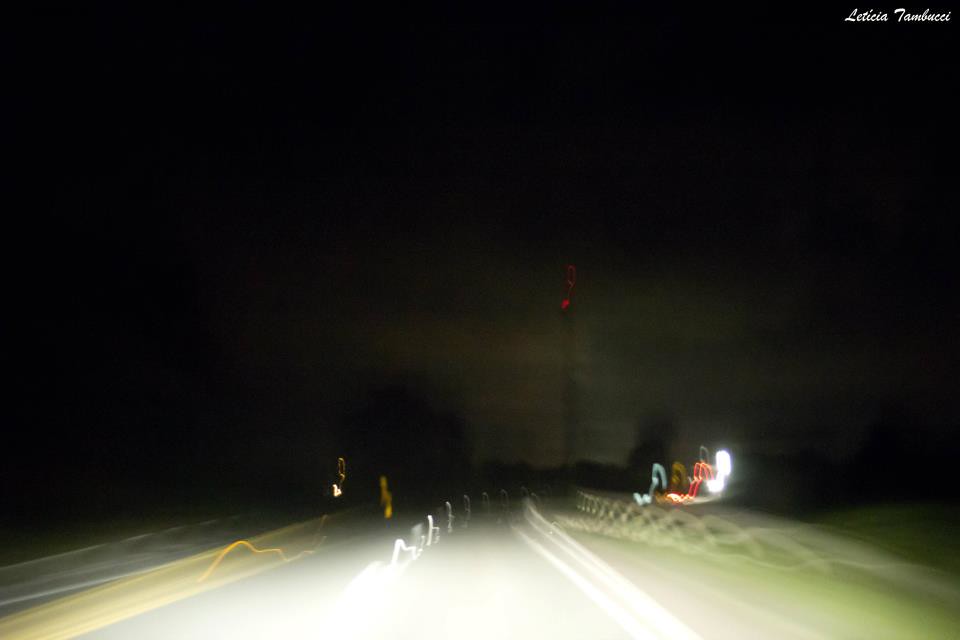This dynamic photograph captures the exhilarating perspective of speeding down a dark highway from within a moving car. The car's headlights pierce through the night, illuminating the road ahead, but creating dramatic distortions in the image. To the left and right, various shapes and lights blur into abstract forms, leaving their exact nature ambiguous. On the right, an indistinct figure might be another vehicle, though its shape is obscured into an unrecognizable blur. The left side features striking light effects, with yellow and white lines blending into the scene. The sense of high speed is palpable, as the distortions and light effects combine to create an almost surreal, disorienting snapshot of night-time driving.